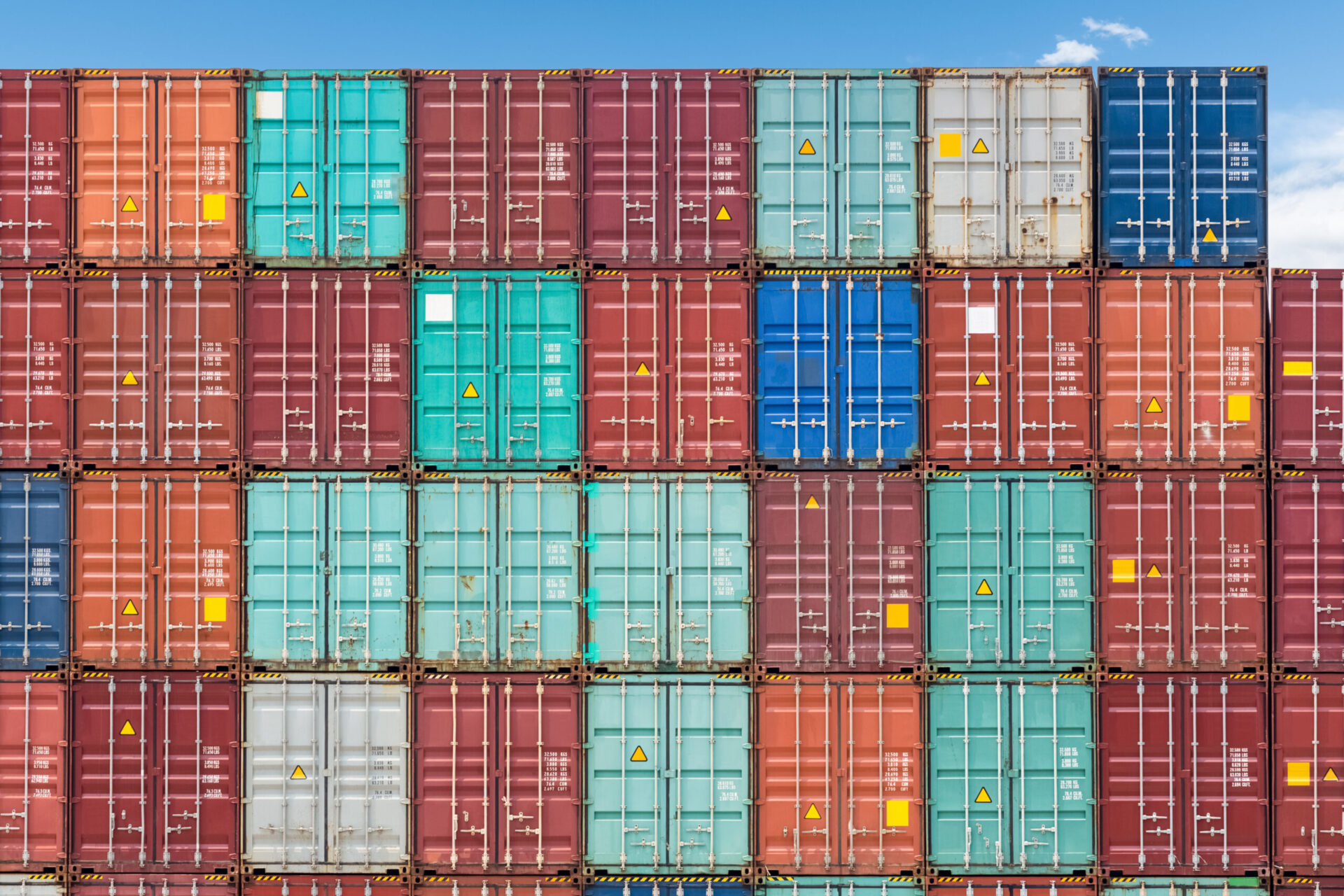The image depicts a highly organized stack of cargo containers, aligned in a tidy grid formation with each container meticulously stacked atop one another, reaching a height of four rows. The containers are predominantly blue, silver, gray, red, teal, green, and orange, and feature white lettering and numbers. Some of them display hazard symbols in yellow triangles, indicating the type of cargo they contain. With at least 25 cargo containers visible, the containers are uniformly rectangular but vary in color. The scene is silhouetted against a clear blue sky with scattered white clouds, providing a backdrop that emphasizes the sheer scale of the stacked containers. Shot head-on as if elevated, the image captures a critical moment at a busy port or shipping location, a space dedicated to the handling and transport of mass freight. Each container is securely shut, with visible handles, and takes up nearly the entire frame, emphasizing the industrial and commercial nature of the scene.